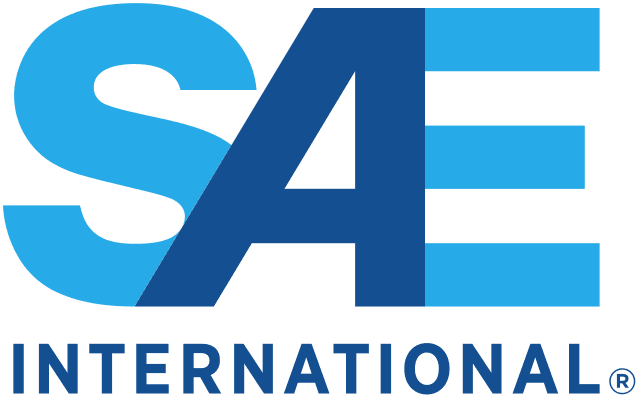In this logo image, against a solid white background, the company name "SAE" is prominently displayed in very large, bold block letters. The arrangement is unique and visually striking: the "S" and "E" are in a lighter shade of blue, while the "A" is in a darker blue. These letters are interconnected — the bottom part of the "S" overlaps with the left side of the "A," and the "E" is formed by three horizontal bars extending from the right side of the "A." Below "SAE," the word "INTERNATIONAL" appears in all-caps, dark blue print. To the right of "INTERNATIONAL," there is a registered trademark symbol, an "R" enclosed in a circle. The design emphasizes the "SAE" text, which is very large and bold, with "INTERNATIONAL" placed underneath in a smaller, yet significant font.